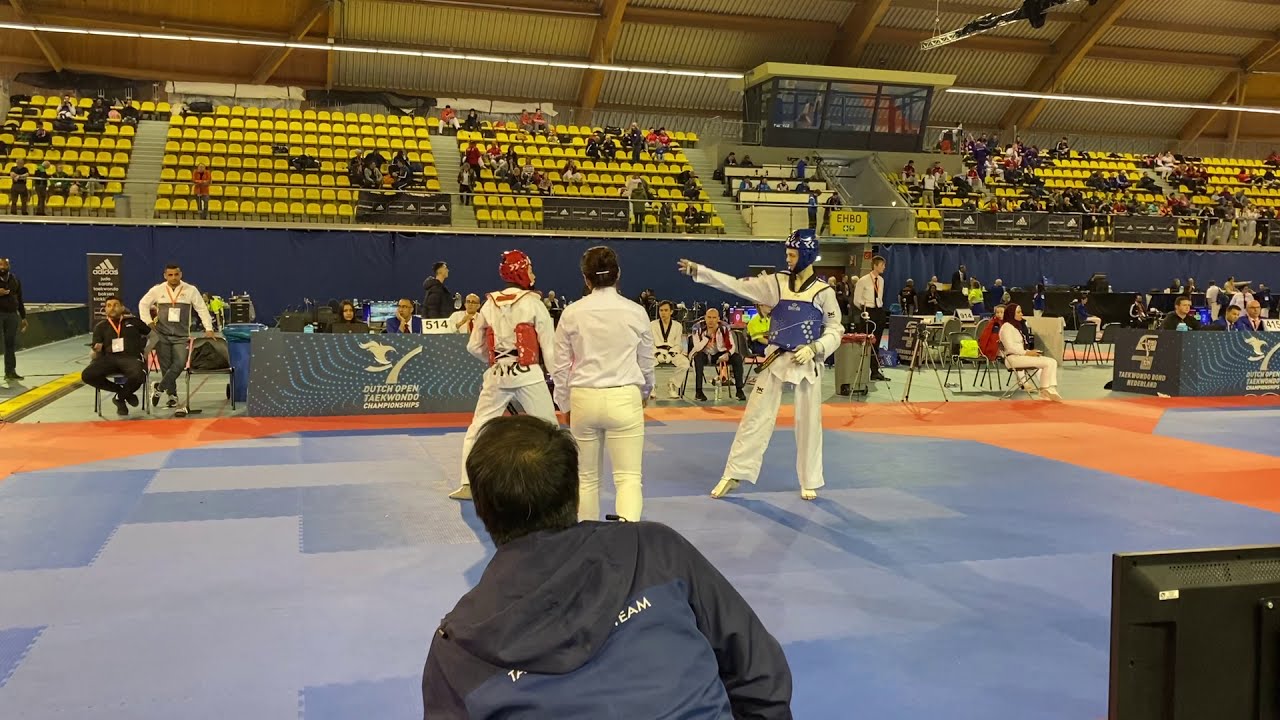The image depicts a Taekwondo match taking place in a large indoor sports arena with stadium-style seating that can accommodate hundreds of spectators, though it appears to be about half full. At the center of the scene, two Taekwondo fighters are positioned on a blue mat. The fighter on the left, whose back is visible, is wearing red protective gear including a helmet and chest guard. The fighter on the right, who is taller and facing the camera, is outfitted in blue protective gear and is extending his right hand towards his opponent. 

A referee, dressed in a light-colored shirt and cream-colored pants, stands near the fighters, overseeing the match. In the foreground, a crouched man with brown hair in a blue jacket appears to be another official or coach. Additional participants and coaches, identifiable by their similar attire, are gathered on the floor next to the fighting area. 

A podium in front of the floor area displays the text "Dutch Open Taekwondo Championships," while another sign in the background includes the words "Taekwondo" and "Netherland" along with various numbers. The audience members are seated in the bleachers toward the back of the arena, attentively watching the match. The overall setting and style of the image is a photograph capturing the dynamic atmosphere of a competitive Taekwondo event.